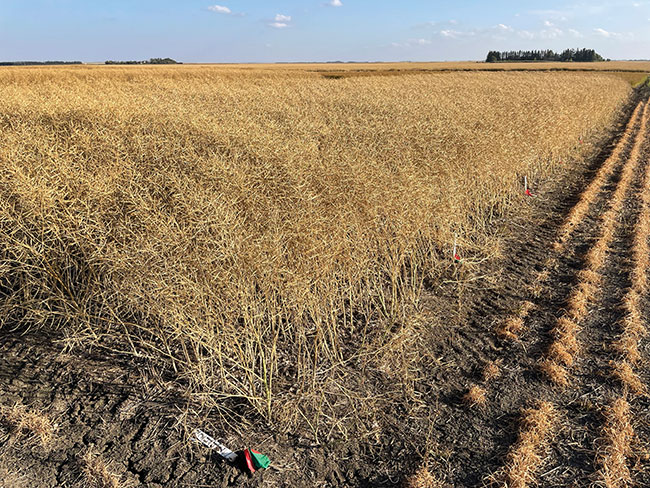This is a detailed photograph of a vast, flat wheat field that stretches as far as the eye can see, covered in golden brown crops, possibly ready for harvest. The foreground features three narrow, straight plowed rows on the right side, with visible indentations likely from a tractor. Among the rows, there are noticeable pieces of trash - a white object and a red and green wrapper. A small, slightly out-of-focus pole with red and green markings stands as a boundary marker. In the lower left corner, a dirt patch breaks the expanse of wheat. Further in the distance, about a mile away, a stand of tall green trees lines the horizon, contrasting against the vivid blue sky with a few scattered clouds, hinting at potential rain. The right edge of the field also showcases another path or mowed area. The entire scene captures the serene and expansive beauty of agricultural land under a partly cloudy sky.